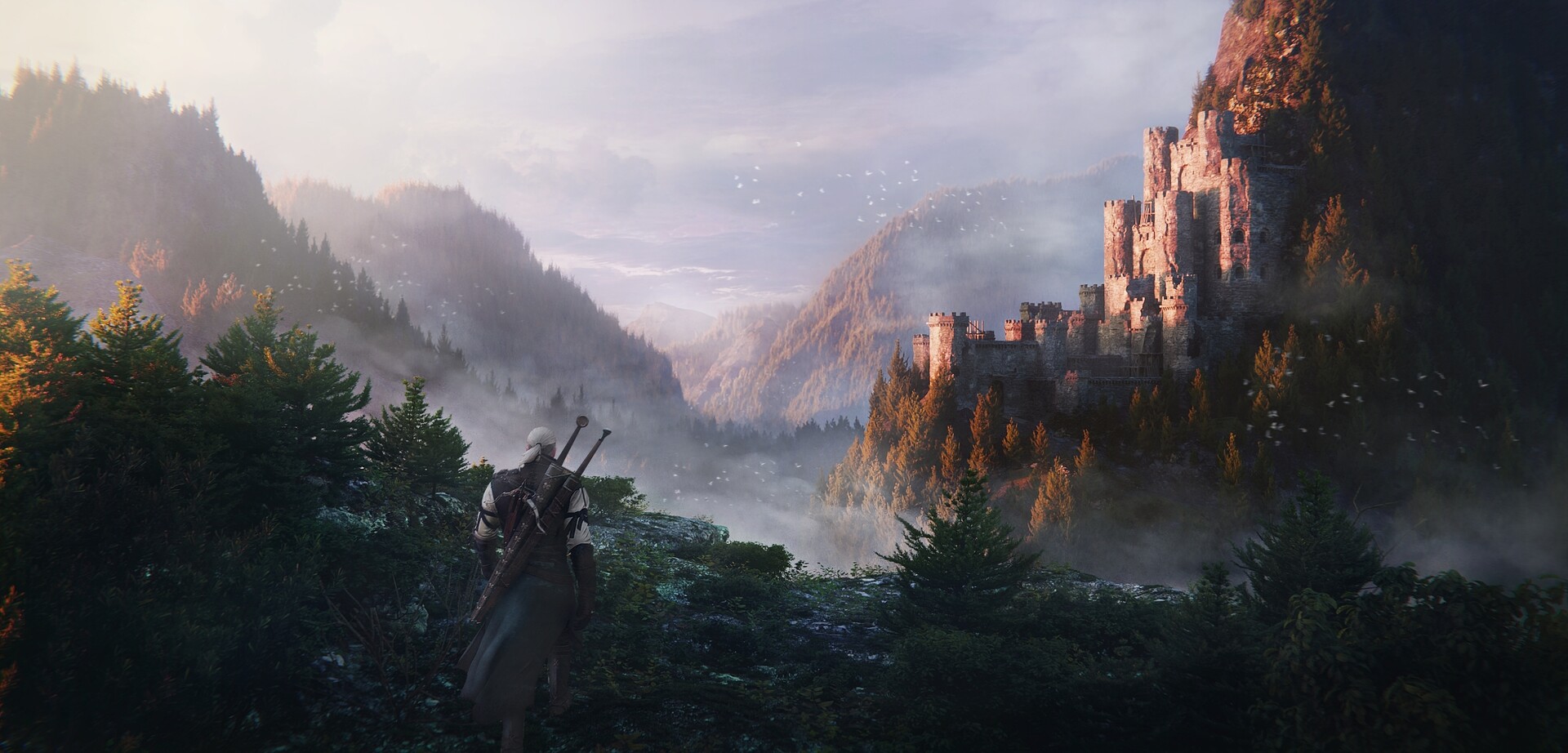This detailed oil painting depicts a city nestled on a mountainside, overlooking a majestic landscape of mountains and forests. The composition features a striking contrast between the dark, almost silhouetted deciduous trees in the foreground and the luminous cityscape bathed in sunlight. A figure, barely discernible among the trees, stands on a cliff's edge. This person, dressed in a mix of black and white with a white helmet, appears to carry either weapons or bagpipes on their back. They blend seamlessly into the darkened foreground, observing the vista.

The city itself dominates the middle right of the painting, perched against the side of a brown, rocky mountain. It's composed of black, white, and gray stone castles, with multiple turrets rising from larger structures. Sunlight streams into the valley, breaking through clouds and mist, casting a golden or orange hue across the city's stone facades, making them look illuminated. The sun's rays also light up the mountain, enhancing its brown and golden tones. In the distance, three or four additional mountains rise under a sky filled with blue and gray clouds, adding depth to the scene. The painting is rich with detail and contrasts, capturing both the serene beauty and rugged grandeur of this mountainous cityscape.